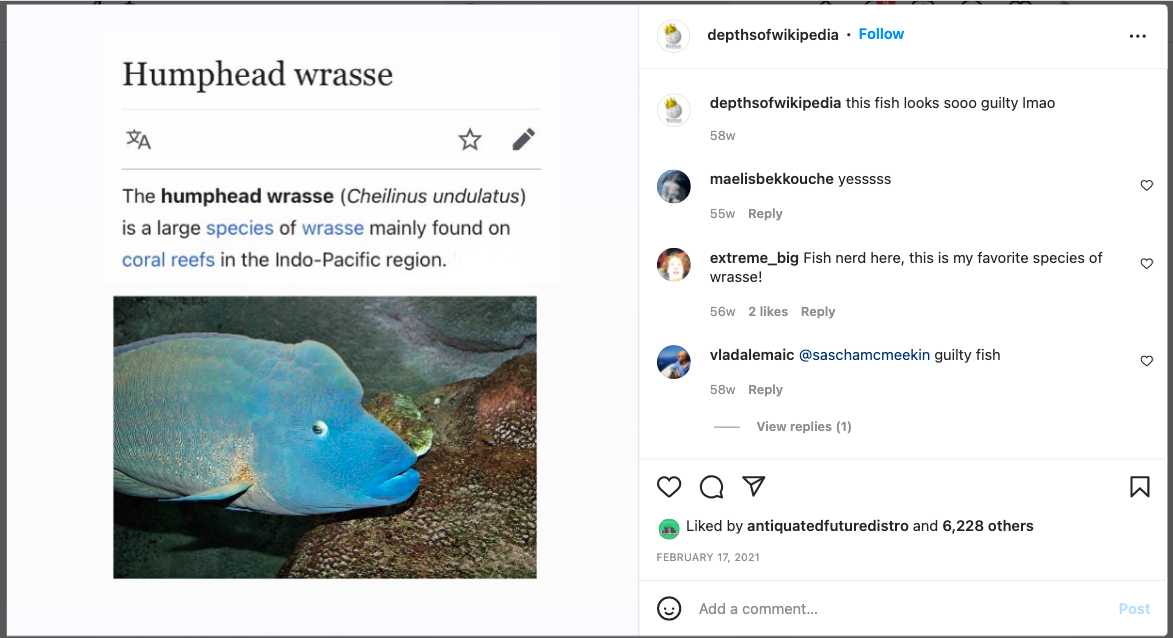The screenshot captures an engaging online discussion about the humphead wrasse. 

On the left side, the screenshot highlights the identification and description of the fish: "Humphead Wrasse" (Cheilinus undulatus). Below the name, there's a translation option, a star for marking the item as a favorite, and an edit button. The explanatory text states that the humphead wrasse is a large species of wrasse mainly found on coral reefs in the Indo-Pacific region. A striking photo of the humphead wrasse accompanies the text, showcasing a vibrant blue fish with thick lips and an almost comical, surprised expression, set against a backdrop of rocks.

On the right side of the screenshot, there's a lively comments section. Users engage with humorous and appreciative remarks:
- "Depth of Wikipedia: This fish looks so guilty, L-M-A-O"
- "yes"
- "big fish nerd here, this is my favorite species of wrasse."
- "guilty fish, the fish does look guilty in fairness."

The timestamps of these comments indicate activity from about 56 to 58 weeks ago. Each comment shows options for replies and likes. 

At the bottom of the screenshot, there are interface options for liking, replying, forwarding, and bookmarking comments. The post has been liked by "Antiquated Future Distro" and 6,228 others, dated February 17, 2021. There's also an arrow to add a new comment.